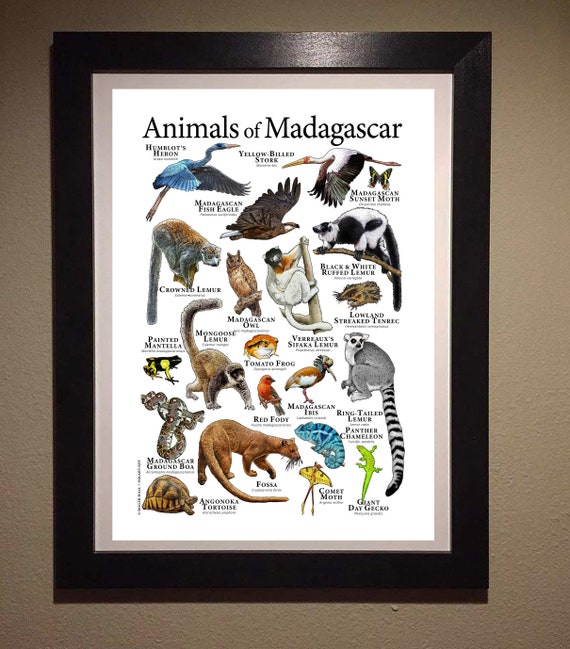This detailed color poster, presented in a tall black frame, hangs on a textured brown wall with a taupe-colored matting. It features a white background with the title "Animals of Madagascar" prominently printed at the top in black ink. Below, the poster showcases an array of detailed illustrations, depicting a diverse collection of Madagascan wildlife. Each animal is meticulously labeled. Among the depicted creatures are:

- Humboldt's Heron
- Yellow-billed Stork
- Madagascan Fish Eagle
- Madagascan Sunset Moth
- Crowned Lemur
- Madagascan Owl
- Black and White Ruffed Lemur
- Lowland Streaked Tenrec
- Painted Mantella 
- Mongoose Lemur
- Tomato Frog
- Verreaux's Sifaka Lemur
- Madagascan Ground Boa
- Red Fody
- Madagascan Ibis
- Ring-tailed Lemur
- Panther Chameleon
- Angonoka Tortoise
- Fossa
- Comet Moth
- Giant Day Gecko 

The poster intricately describes each animal, contributing to an informative and visually engaging representation of Madagascar's rich biodiversity.